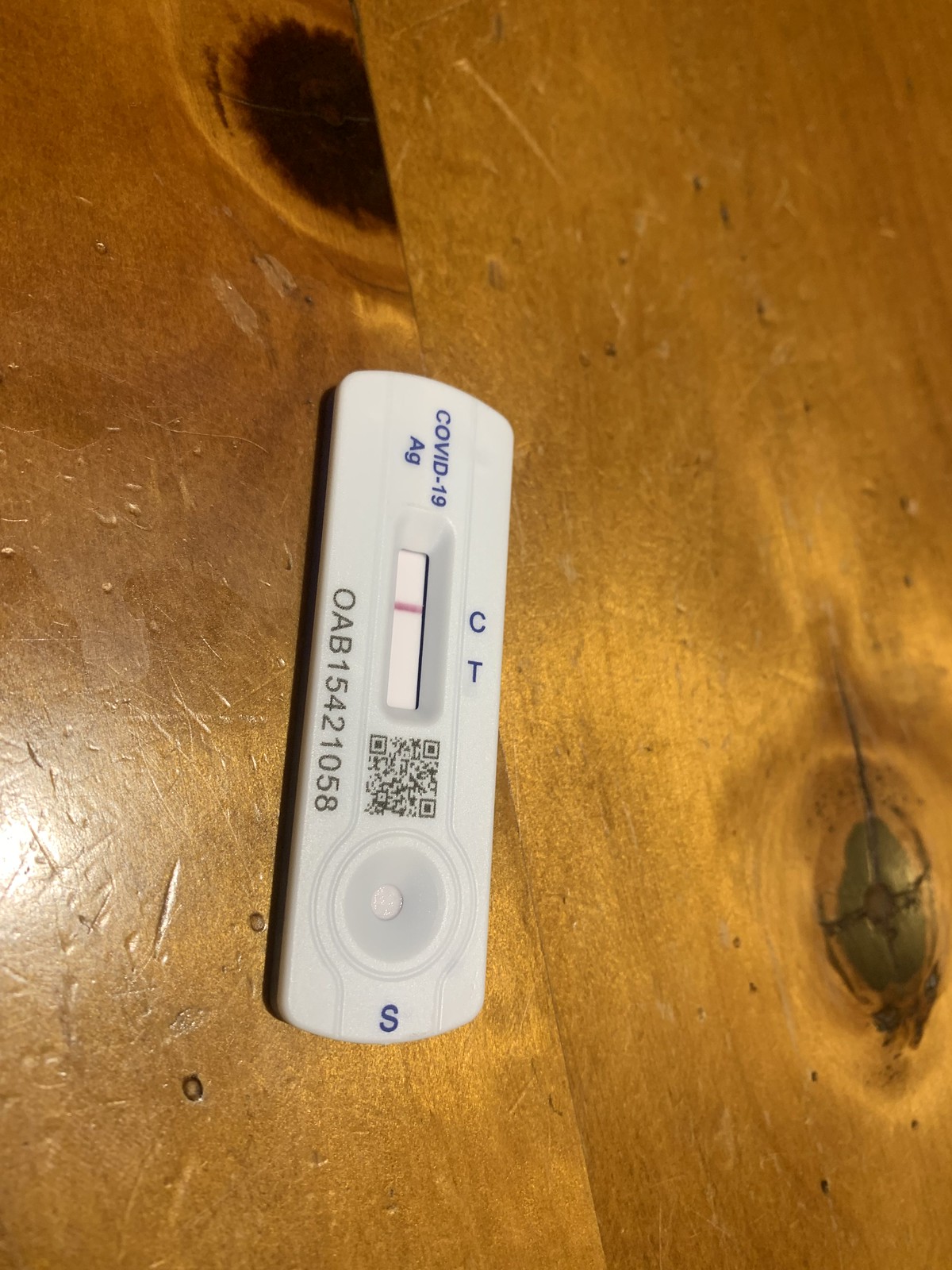This image features a COVID-19 rapid antigen test kit. The test is encased in a white plastic device, characterized by a central display screen. At the top of the device, the label "COVID-19" is prominently displayed in blue, set at a slight angle. Below this label, the letters "AG" are indicated. In the middle of the screen, there is a horizontal red mark extending across, aligning on the right side with the letter "C." Directly beneath the "C," the letter "T" is marked. Below the display screen, a QR code is visible, followed by an indentation on the device. The entire apparatus rests on a wooden table.